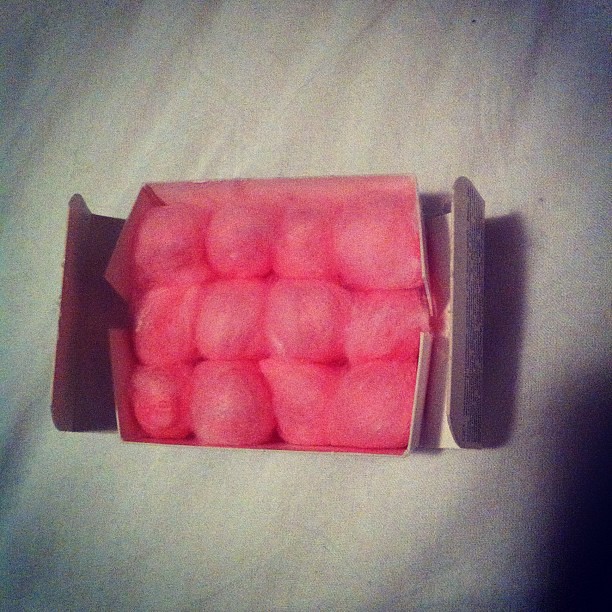The photograph is a close-up, slightly out-of-focus indoor shot showcasing an open cardboard box on a white background. Inside the box are 12 pink, slightly fuzzy-looking objects, arranged in three rows of four. The objects are not perfectly round and appear to have been shaped by hand, resembling the texture of cotton candy, or possibly resembling hairy or yarn-like qualities due to the graininess of the photo. The pink coloration of the objects is slightly darker than cotton candy, akin to the shade of Pepto-Bismol. The box, which has some fine print that's difficult to discern, casts a slight shadow to the right, indicating lighting from the left. The overall image quality is slightly blurry, adding to the mystery of what these pink items might be.